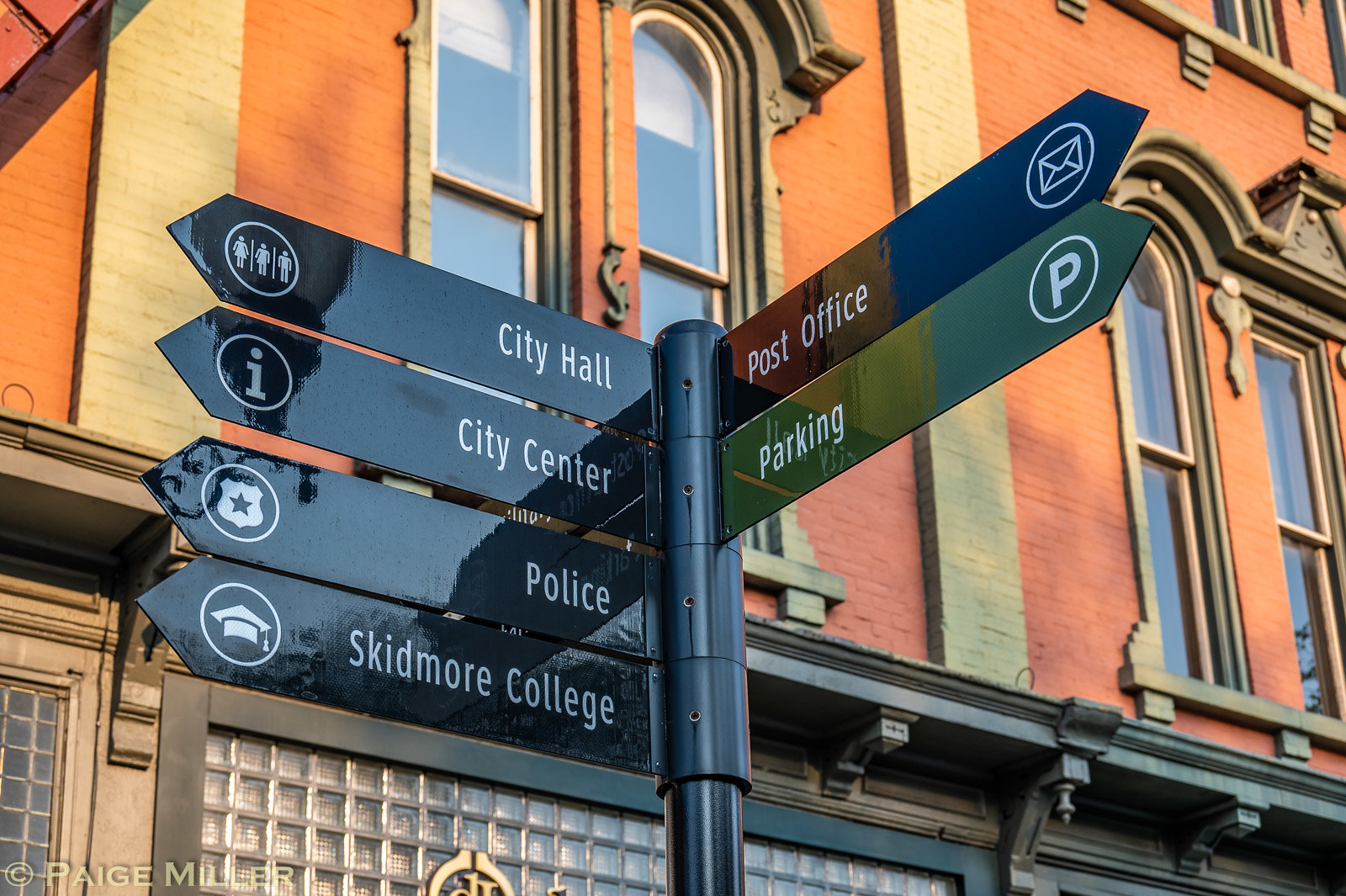This outdoor city scene features a prominent black cylindrical metal direction post with multiple horizontal metallic arrows extending from the top, each adorned with white text pointing towards various locations. To the upper right, the first arrow directs to the post office, marked with a circular symbol of a letter; below it, a lime-green rectangle indicates parking with a 'P' in a circle. Pointing to the left are four similarly styled, dark blue arrows with white text and unique symbols: City Hall (three figures), City Center (an information 'i'), Police (a badge), and Skidmore College (a mortarboard).

Behind the signpost stands an older, multi-story building with a mix of orange and yellow bricks. It features ornate, arched and sash windows, and glass block windows at the base. In the lower left corner of the image, there is a faint watermark reading "PAIGE MILLER" with a copyright symbol. The composition of the photograph emphasizes the clean, shiny metallic street signs and the historic architectural backdrop, captured with a slightly upward angle.